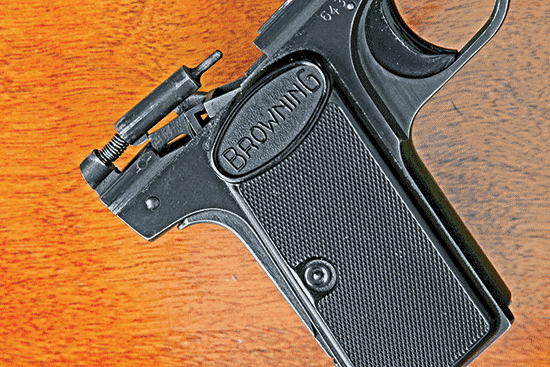The photograph captures a black Browning pistol resting on an orange-ish brown wooden surface with darker wood grain accents. Only part of the firearm is visible, mainly the grip and the back, with the front cropped out of the frame. The image, oriented horizontally, reveals the gun's rectangular, textured grip, which is tilted with the handle pointing up and to the left. Prominently displayed on the grip is an oval frame containing the raised text "Browning." In the upper right corner, the black loop-shaped trigger is visible. The top portion of the pistol appears to be missing, exposing internal components, including a cylindrical firing pin and a coiled spring in the back, with a small striker piece adjacent to it.